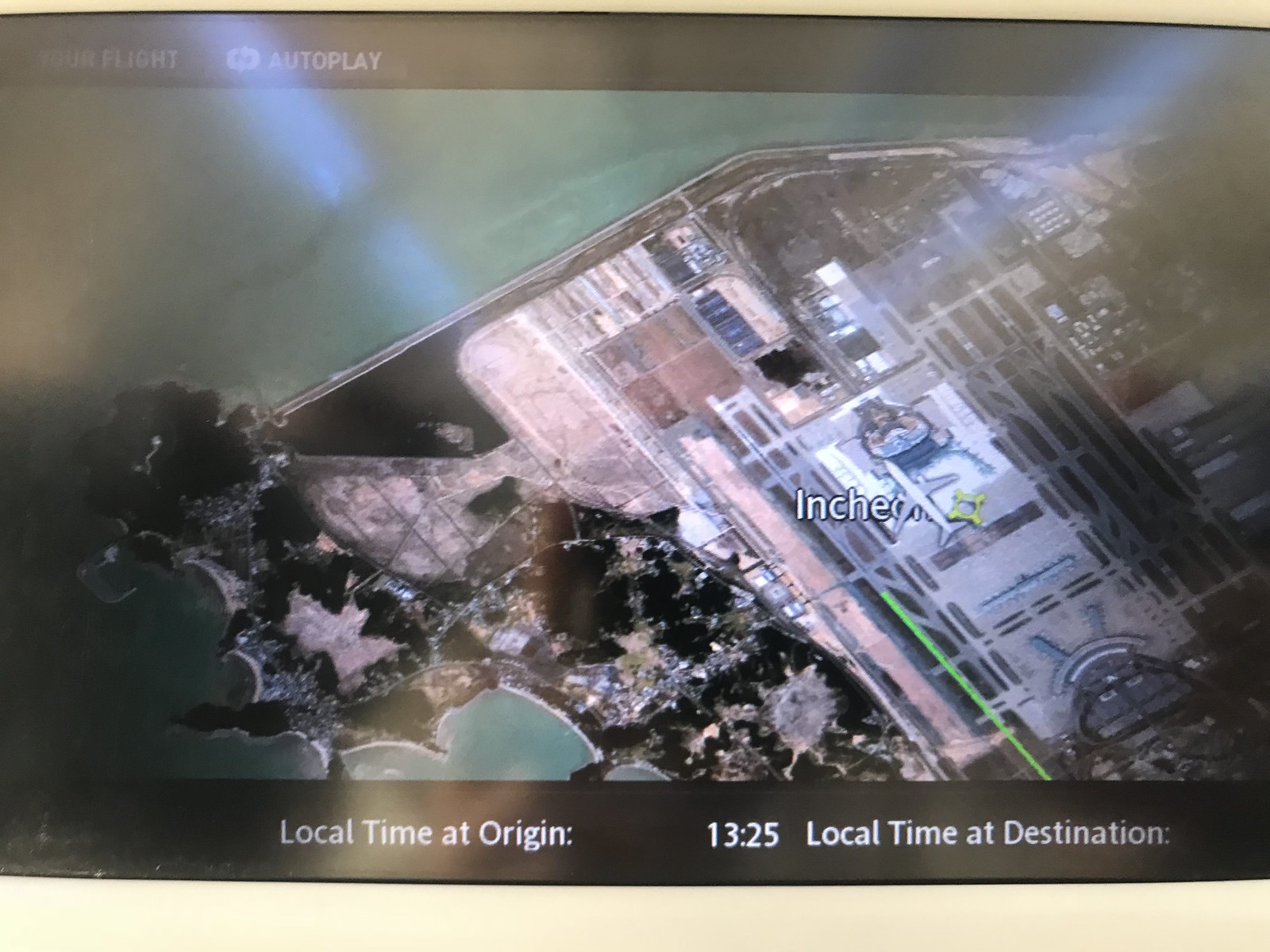This image is a screenshot of a flight information display on the back of an airplane headrest. The screen shows an aerial view, likely a satellite image, of an airport centrally framed. A white airplane with gray wings is prominently visible at the center, next to a yellow circle with dots on its corners. Below the airplane, the word "INCHED" is displayed. The airport layout features a circle with runways on both the left and right sides, with a light green line extending from the bottom right to the top left, indicating the flight path or trajectory. The upper part of the screen has a green-black strip displaying the words "FLIGHT AUTOPLAY" with a heavy shadow and light blue streaks of reflection. The bottom black bar shows the text "local time at origin 13:25" while the destination time is partially cropped off.